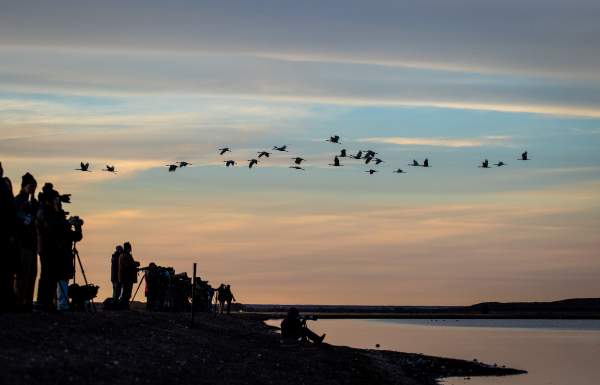This evocative photograph, taken from a distance, captures a group of silhouetted photographers gathered on a shoreline at twilight. The scene is bathed in the soft hues of a dusky sky, where thin, horizontal clouds stretch across the horizon, subtly illuminated by the setting sun. To the right, a calm body of water reflects the tranquility of the evening.

In the midground, a bank ascends about 10 to 12 feet from the water's edge, where an array of people equipped with tripods, DSLR cameras, and other sight devices are intently focused on the sky. They appear to be observing or photographing a flock of large birds, possibly ibises, egrets, or ducks, flying in a distinctive formation. The entire scene is cast in a shadowy silhouette, emphasizing the striking contrast between the darkened figures and the gradually darkening, colorful sky that transitions from a light blue near the middle to darker, pinkish tones near the horizon and bottom of the image.

The overall atmosphere of the photograph is serene, capturing the intersection of nature's grandeur and human curiosity in a beautifully composed snapshot of a twilight moment by the water.